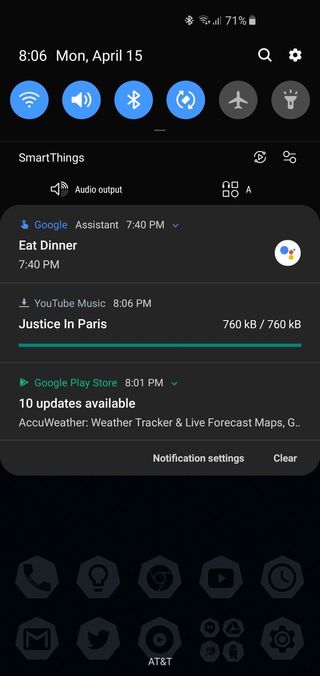The image depicts a smartphone screen with a detailed interface. The screen is mostly black, with various white and blue icons scattered throughout.

1. **Top Status Bar**:
   - **Right Side**: Shows a 71% battery icon, signal strength bars, and a volume icon, all in white.
   - **Left Side**: Displays the time "8:06", the day "Monday, April 15th," and a white search bar with a white settings icon adjacent to it.

2. **Quick Access Toolbar with Six Circles**:
   - The first four circles are blue:
     1. The first blue circle contains a white half-circle, possibly representing volume control.
     2. The second blue circle features a white bell symbol, likely for notifications.
     3. The third blue circle has a white ribbon-like icon, the exact function is unknown.
     4. The fourth blue circle shows an arrow pointing up and down with a square in the middle, presumably for screen rotation.
   - The last two circles are gray:
     1. One gray circle contains an airplane icon, representing airplane mode.
     2. The other gray circle displays a flashlight icon.

3. **Main Screen Content**:
   - The left side features "Smart Things" and an audio output section, possibly indicating connected devices or apps.
   - On the right side, there are four tiny icons: headphones, a square, a square with a circle, and a gray icon with an 'A'.
   - The central area has a gray shaded section with "Google" in blue and "Assistant" in white.
     - Below it, there's a time display "7:40 PM" next to a blue-downward arrow and an "Eat Dinner" reminder.
     - It shows a white circle with Google-colored dots, likely a calendar event marker.
   - Notifications:
     - A "YouTube Music" notification at 8:06 PM, with the mention of "Justice in Paris," and file sizes "760KB - 760KB".
     - A "Google Play Store" notification at 8:01 PM with a green arrow, indicating "10 updates available."
     - The weather tracker app "AccuWeather" and the word "notification settings" at the bottom along with an option to "clear."

4. **Bottom Dock**:
   - Consists of two columns each featuring five icons in octagonal shapes:
     - **First Column**:
       1. Telephone
       2. Lightbulb
       3. An unknown icon with a black circle and lines
       4. Possibly the YouTube logo with a square and arrow
       5. A clock with hands
     - **Second Column**:
       1. Gmail with a black square and white 'M'
       2. Twitter bird
       3. A video-related icon with a black circle and white elements
       4. Two dots in a black circle (exact purpose unclear)
       5. A triangle with small adjacent arrows

5. **Bottom Right**:
   - A black settings icon and the carrier name "AT&T."

The overall interface is dense with various icons and notifications, offering a range of functionalities and quick-access features to the user.